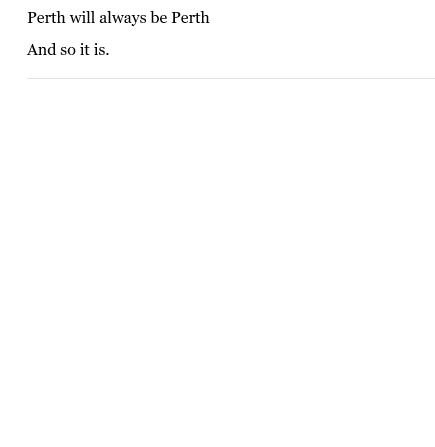The image presents what appears to be an excerpt from a digital or online book, possibly a quickly typed section from a document. At the top left of the image, the first line reads, "Perth will always be Perth," followed by the second line directly underneath, "and so it is." Below these lines, a thin, gray, horizontal separator stretches across the width of the image, adding a subtle division between the textual content and the rest of the document. The simplicity and minimalism of the layout draw attention to the poignant, repetitive message concerning Perth.